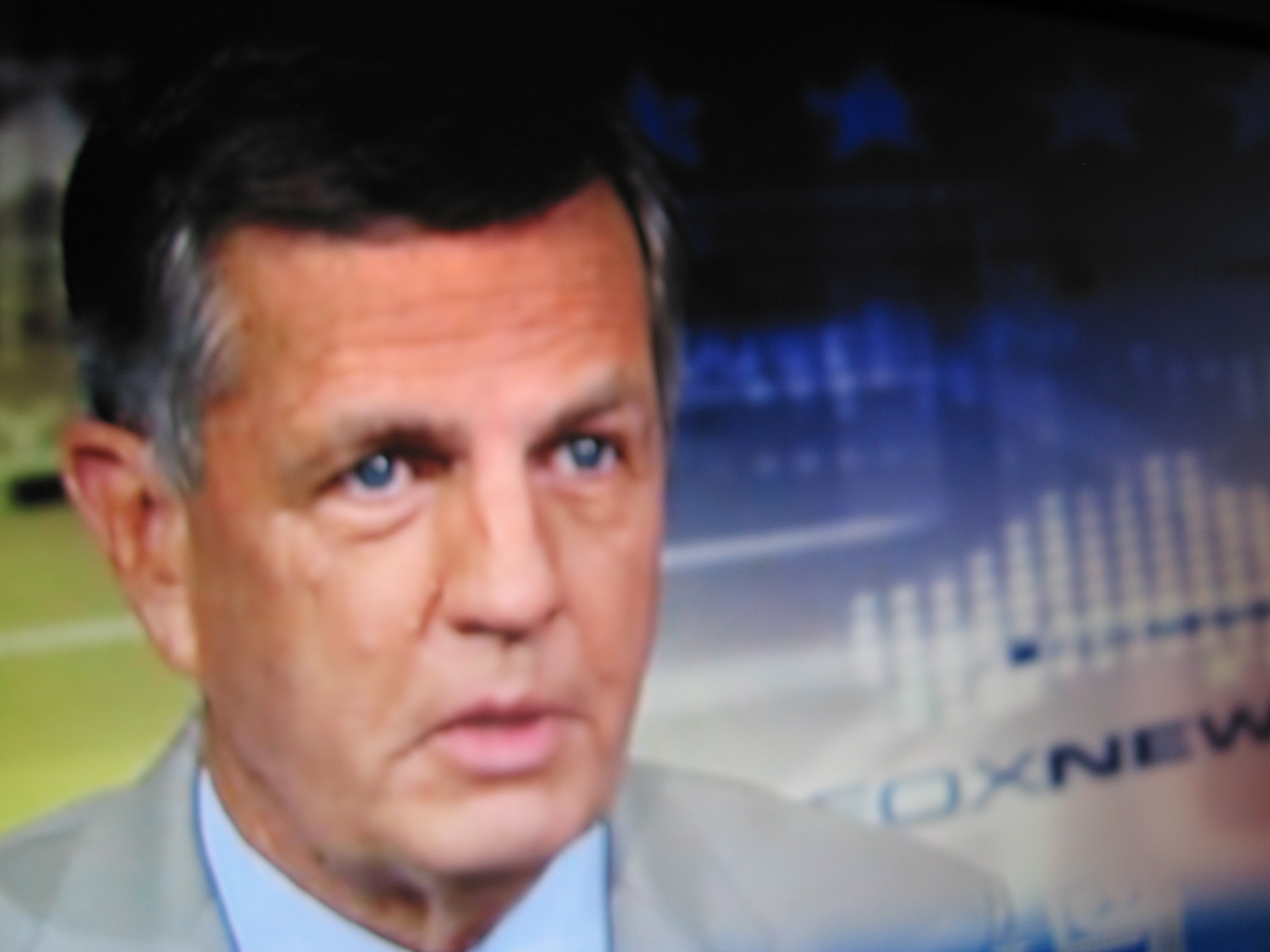The image appears to be a blurry screen grab taken from a TV screen, depicting a post or pre-match event with Fox News coverage. In the background, there is a logo of Fox News and an indistinct screen showing what seems to be a field or ground, alongside some abstract colors—yellow to the left and black and blue to the right. The central figure in the image is a middle-aged to older white man with salt and pepper short hair, blue eyes, and clean-shaven. Only his face and part of his shoulder are clearly visible. He is wearing a gray suit over a black-blue shirt and appears to be speaking directly to the camera.